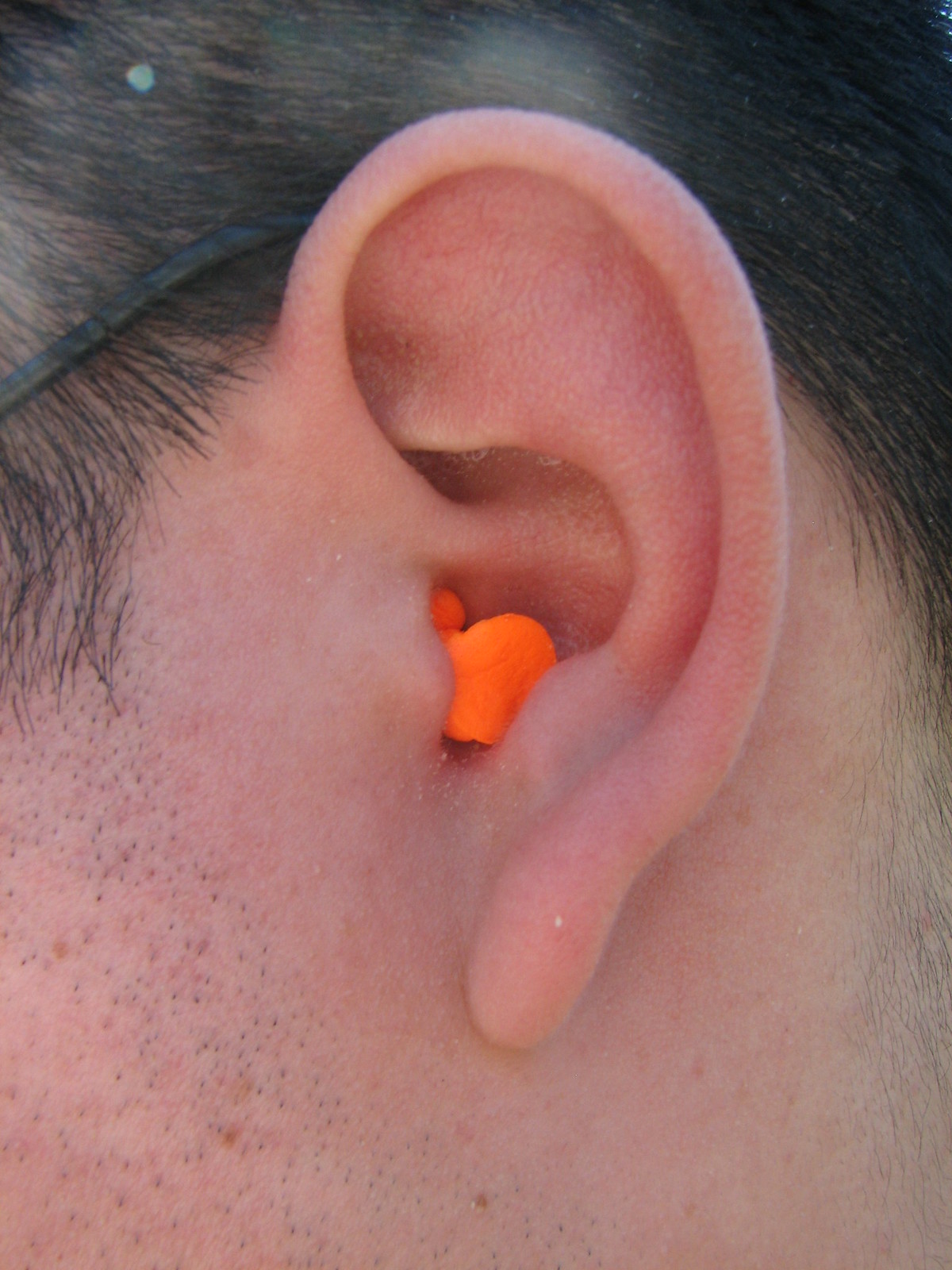This is an extreme close-up of a man's ear, positioned centrally in the image. The man has short brown hair, cleanly cut around the ear. A black arm of his glasses extends behind his ear, curving down the left side. Prominently featured in the ear is an orange earplug, likely for noise protection. Fine, faint stubble is visible where his sideburns would be, indicating he hasn't shaved in about a day. The zoomed-in perspective reveals slight whitish crusty areas inside the ear, and subtle marks of shaving and dark pores along the sideburns. The overall focus of the image is clearly on the orange earplug nestled in his ear.